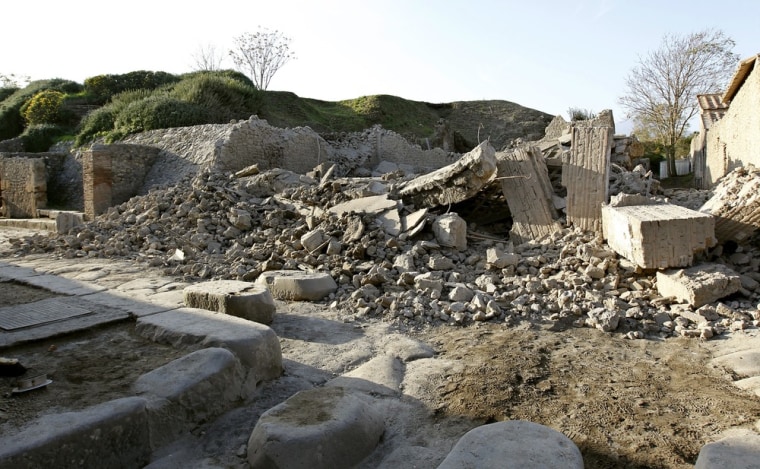The image depicts a post-demolition scene where a once-standing building has been reduced to a sprawling pile of rubble. To the left, a visible foundation is littered with large stones, suggesting the starting point of the structure. Straight ahead, the ground is strewn with heaps of bricks, broken stones, and sizable chunks of stone slabs. Scattered among the debris are sections of bricks still adhered together, hinting at the original construction's robust nature. In the distance, partial remnants of the building’s walls stand precariously, including a partially complete brick wall on the far left. To the right, a relatively intact building looms in the background, contrasting sharply with the destruction in the foreground. A leafless tree stands straight ahead, adding a somber touch to the scene, while a hilly green area extends into the background. The foreground features a blend of dirt patches and segments of pavement, completing this vivid snapshot of the aftermath.